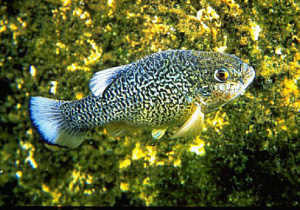The image features a small, visually striking fish swimming in the ocean against a backdrop of dark green to white coral or rock formations. The fish's body is predominantly silver-white, adorned with a complex, maze-like pattern of black squiggles. Its gills and several fins on either side of its body are also white. The tail fin stands out with a white center bordered by a black outline and blue fringes. The fish is oriented facing to the right, with one eye gazing directly at the camera. The scene captures the fish in its vibrant underwater habitat, contrasting sharply with a very dark area in the bottom right corner of the image.